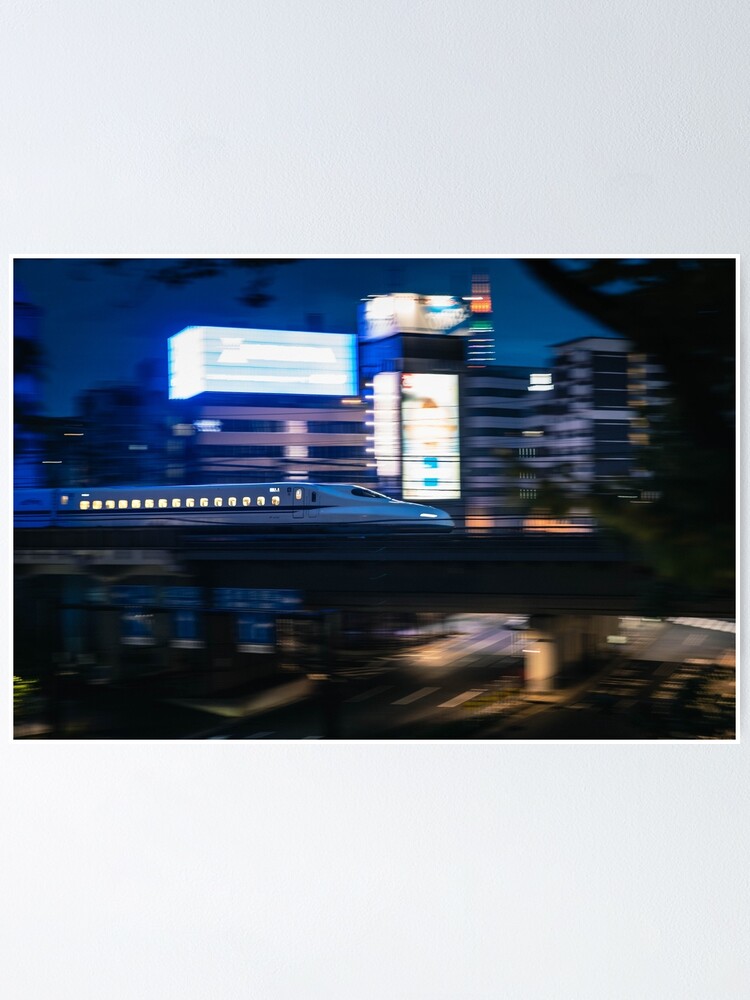The image showcases a heavily blurred, possibly computer-generated city scene at dusk, dominated by a horizontally oriented white monorail train with a sleek, torpedo-like design. The monorail, illuminated with yellow lights through its windows and displaying a small cockpit windshield on the front right side, traverses a bridge supported by concrete columns. Below the bridge lies a roadway, with visible lanes divided by a buttress. To the right of the monorail, a green-leafed tree extends from the edge of the image. The background features multiple city buildings, including some with dark windows and various colorful neon signs, particularly blue and yellow, atop and on the sides of the structures. Above these buildings, the darkening blue sky is tinged with dark clouds, adding to the nighttime ambiance.